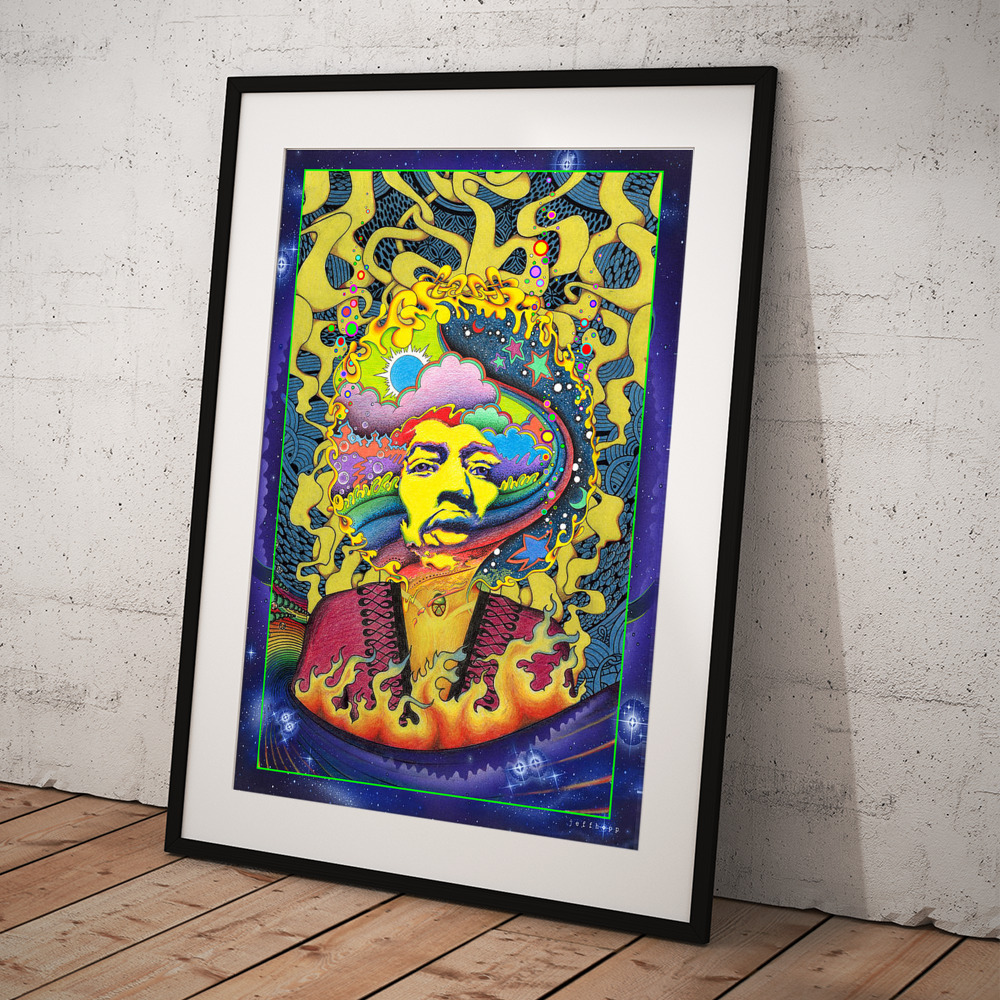This photograph captures a framed psychedelic artwork of Jimi Hendrix, leaning against a white, painted brick wall with detailed pale wooden floorboards beneath. The image is housed in a black frame with a thin black border and features a white matting. The artwork itself is vibrant, with a blue and purple background highlighting Jimi Hendrix, rendered in a highly psychedelic style. His hair transforms into rainbow tones interwoven with clouds, flames, stars, and starfish. Above him, a swirling yellow ribbon adds to the surreal atmosphere. Flames, depicted in yellow and orange with hints of blue and grey at the tips, surround his chest, suggesting intense heat. He is depicted wearing a pink top adorned with black embroidery. This artwork, evocative of the 60s psychedelic era, brilliantly captures the essence and mood of Jimi Hendrix.